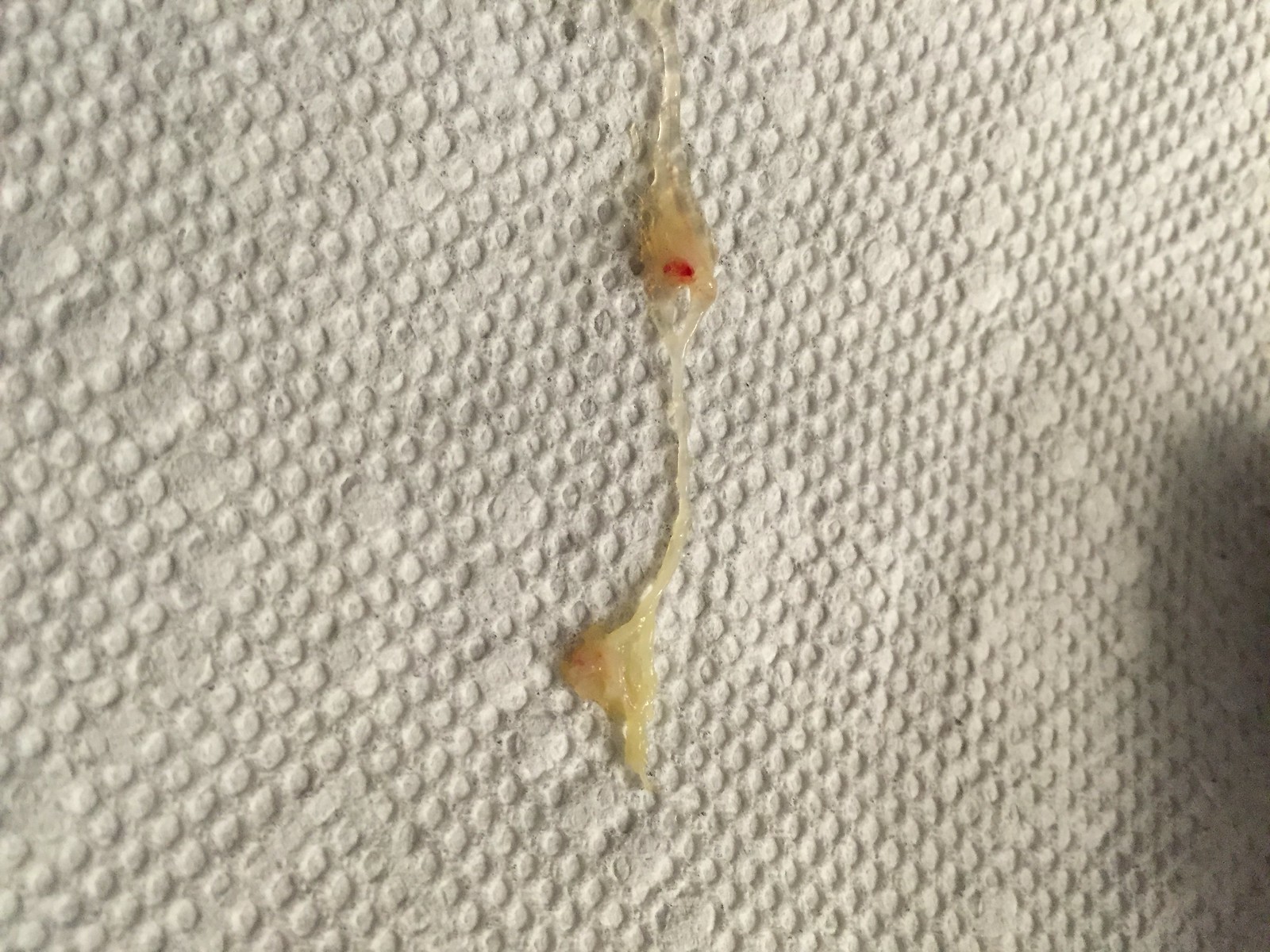The color photo captures a highly detailed close-up of a white, quilted paper towel with a distinctive pattern of raised dots forming curved figures and a diamond shape in the center. Laid across this textured surface is a long, stringy, and somewhat disgusting glob of snot. The upper portion of the snot is particularly notable, featuring a thick, chunky consistency with whitish elements interspersed with blood. Moving down the snot trail, the texture transitions to a more stringy, clear substance, eventually becoming a thick, yellowish, dried gunk towards the bottom. Additionally, some blood appears along the left side of the napkin. The scene is illuminated from the left, casting subtle shadows and causing a slight darkening at the bottom right, adding to the overall gritty and unappealing aesthetic of the image.